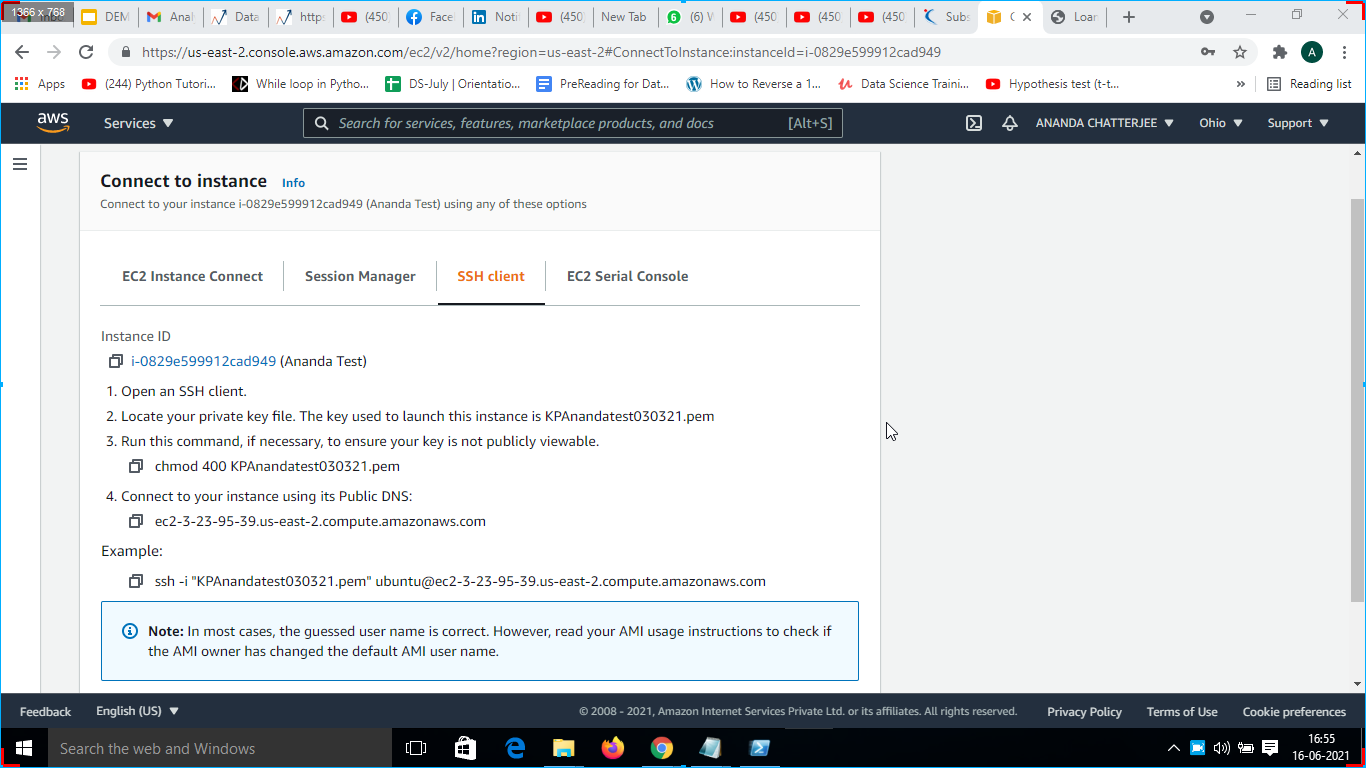A detailed screen capture displaying a multitude of browser tabs and a variety of color-coded elements:

At the top of the capture, the browser's tab bar is visible, featuring approximately 20 open tabs. Among these, there is a gray-colored tab labeled "DEM", a Gmail tab, two tabs with small graph icons, a red YouTube tab, a Facebook tab, a LinkedIn tab, and another YouTube tab. Additionally, there's a button marked "New Tab", a gray and green circle icon tab, three more YouTube tabs, a tab partially labeled "SUB", featuring a blue and red graphic, a gold box tab, and a tab with a gray globe icon.

To the top right of the browser, typical navigation and control icons are present. These include a plus sign, a gray circle, minimize/maximize/close (X) buttons, a back arrow, a grayed-out forward arrow, a refresh button, and an address bar featuring a padlock icon. Accompanying this bar are a key icon, a star icon, a puzzle piece icon, a dark, forest green circle with a white "A" in it, and three gray dots.

Further down the page, the main visible content appears to be a YouTube page titled "Python tutorial". Alongside are various icons: a black icon with partial white text "loop ... Python", a green icon with a white cross labeled "DS July orientation", a blue icon titled "pre-reading for ...", and a blue circle with a white "W" labeled "how to reverse A1 ...". 

Additional visible tabs include a red "U" labeled "data science training ...", another YouTube tab titled "hypothesis test ...", and a newspaper icon labeled "reading list".

Moving downward, there is a gray bar with text "AWS" followed by the Amazon smiley logo. The menu includes options for "Services", a pull-down menu, a search box for searching services/features/marketplace/products/docs with a keyboard shortcut suggestion "Alt + S". On this toolbar are various icons: a box, a bell, an avatar with "it", a chat tree, pull-down menus labeled "Ohio" and "Support", and options related to EC2 instance management including "EC2 instance connect", "Session Manager", "SSH client", and "EC2 serial console", all accompanied by strings of alphanumeric data for configuration.

At the bottom of the image is a dark navy strip with site-related text, including "Feedback", "English US", "2008 to 2021 Amazon Internet Services Pvt. Ltd. or its affiliates. All rights reserved. Privacy Policy Terms of Use Cookie Preferences". Beneath this is a black bar containing text "Search the web and Windows" with icons for a phone, shopping bag, Internet Explorer, file folder, Firefox, Google Chrome, Notepad, computer desktop, a white triangle, a blue and white box, a speaker, and a text bubble. The date displayed at the bottom indicates "May 16, 2021".